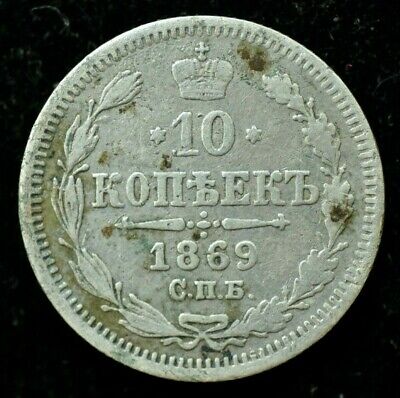This professional photograph showcases an antique silver coin prominently set against a mostly black background with subtle marbling and white imperfections. The coin, displaying signs of greenish decay or oxidation, features intricate designs. At the top, a crown with a cross is encircled by a wheat leaf pattern forming an almost-complete circle around the coin. Below the crown, the coin is marked with the number "10" flanked by two star shapes. An undecipherable inscription follows, potentially in Cyrillic or a similar foreign script, suggesting the coin is of non-English origin, possibly Russian or from a former Eastern European nation. Further down, the date "1869" is inscribed, indicating this coin is over 150 years old. The outer rim features jagged, gear-like edges, adding to its unique aesthetic. This professionally captured image highlights the coin's historical and numismatic significance.